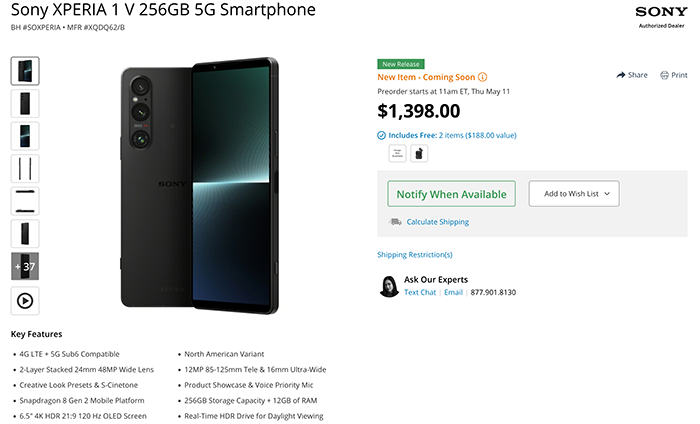The image features a detailed advertisement for a new Sony smartphone. In the upper right corner, the Sony logo is accompanied by the text "Authorized Dealer." Below this, there is a product code composed of a complex string of letters and numbers. The central portion of the advertisement prominently displays an image of the phone.

Underneath the phone image, a list of key features is provided:
- GLD and 5G sub-6 compatible
- 2-layer stack
- 24mm, 48MP wide lens
- Creative look presets in 5S Syntone
- Snapdragon 8 Gen 2 mobile platform
- 6.5-inch 4K HDR screen with a 21:9 aspect ratio and 120Hz OLED display
- North American variant
- 12MP, 85-125mm ultra-wide lens
- 256GB storage and 12GB RAM
- Fast eHP and real-time HDR drive for daylight viewing

A green box indicates this is a "New Release," and nearby text mentions, "New item coming soon" with the date Thursday, May 11th. The price is listed at $1,390. Below this, a message offers "Free 2 items," and a green button labeled "Notify Me When" is next to a grey button labeled "Add to Wishlist," featuring a downwards-pointing arrow. Further down, options for calculating shipping costs and noting shipping restrictions are provided. Finally, there is an invitation to "Ask Our Experts," repeated twice for emphasis.